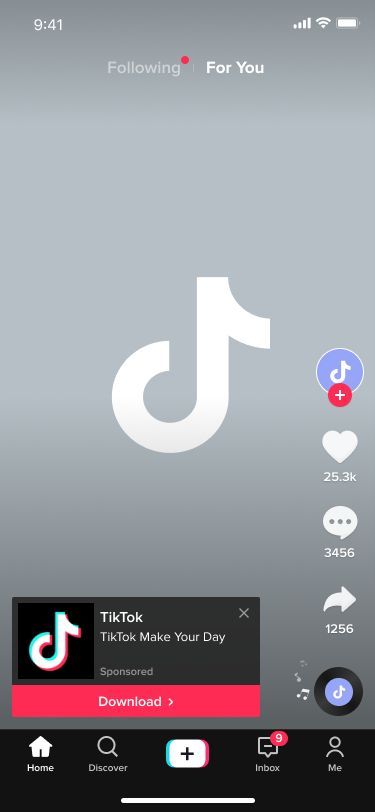This detailed caption encapsulates the complexity of the TikTok screenshot, including specifics about the content and the interface:

"A screenshot taken at 9:41 AM shows a TikTok loading page. The phone displaying the screenshot has fully charged battery and full cellular data bars, indicating a strong connection. The user is also connected to Wi-Fi. The TikTok screen has a gray background adorned with a large TikTok logo in the center, and a smaller TikTok logo at the bottom. The text on the screen reads: 'TikTok, TikTok, make your day, sponsor, download now.' The TikTok interface layout is evident, showing options to like, comment, or share, as well as icons for accessing TikTok audio, home screen, discovery page, record (plus button), inbox, and user profile (me). The download button is prominently displayed in red. It appears to be a loading page since no specific video content is visible."